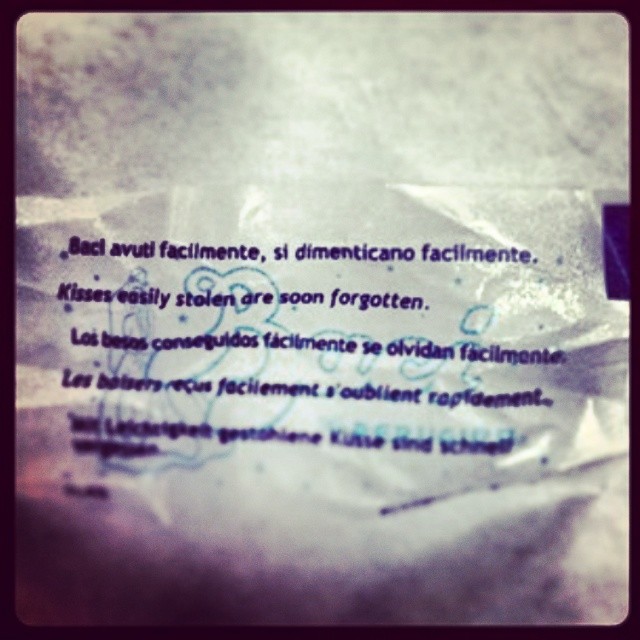The image depicts a crinkled, wrinkly piece of paper or possibly cellophane, which has writing in five different languages. The paper appears to be laminated in plastic, reflecting a certain sheen. It's placed against a rough, grey background, potentially a table or a sidewalk, and is framed by a black border. The writing includes one English sentence that reads "Kisses, easily stolen, are soon forgotten." The first sentence begins with the word "Baci" which is Italian for kisses. The last sentence, difficult to decipher, seems to include a word resembling "K-U-S-S-E." There are three additional lines of text, one of which splits into a sixth line. The text is in dark ink, either black or dark blue. A light blue, almost graffiti-like watermark featuring the word "Baci" and a small cartoon or drawing is subtly visible in the background.